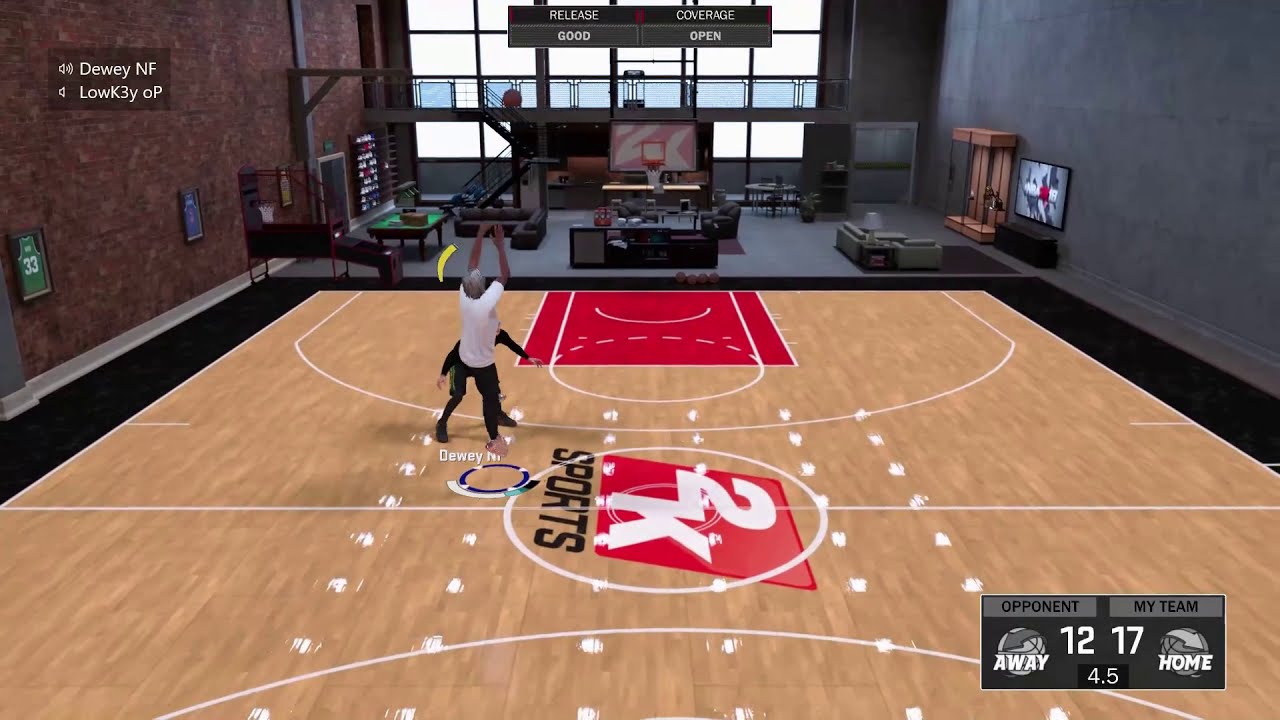The image captures a scene from a basketball video game by 2K Sports. The court, with its wooden floor and black border, features the red 2K Sports logo at its center. The free throw area is marked in red. The game environment seems to be set in a gym or possibly a mansion, suggested by its detailed backgrounds. 

On the left side, the wall is made entirely of red brick, adorned with framed basketball jerseys. The right wall is a gray-black metal surface with a mounted TV and possibly a trophy case or display area beneath it. Below the court, closer to the viewer, one player named Dewey N-F, as indicated by the top-left name tags, is jumping up to shoot a basket. Dewey is wearing a white shirt, gray hat, and black pants. The opposing player, Lowkey O-P, remains grounded, dressed in black pants and a shirt.

Beyond the basketball court, the background depicts a studio-like setting with multiple TV screens, chairs, and brown doors on the right. There's also a desk in the middle and a sofa on the right wall facing another TV, with a hoop in the foreground. The left wall of the court lacks seating for an audience and is entirely blank. The bottom right of the screen shows the score: the opponent has 12 points, and "my team" leads with 17 points, with a game time of 4.5 minutes displayed below. Circles indicating "away" and "home" teams flank the score.